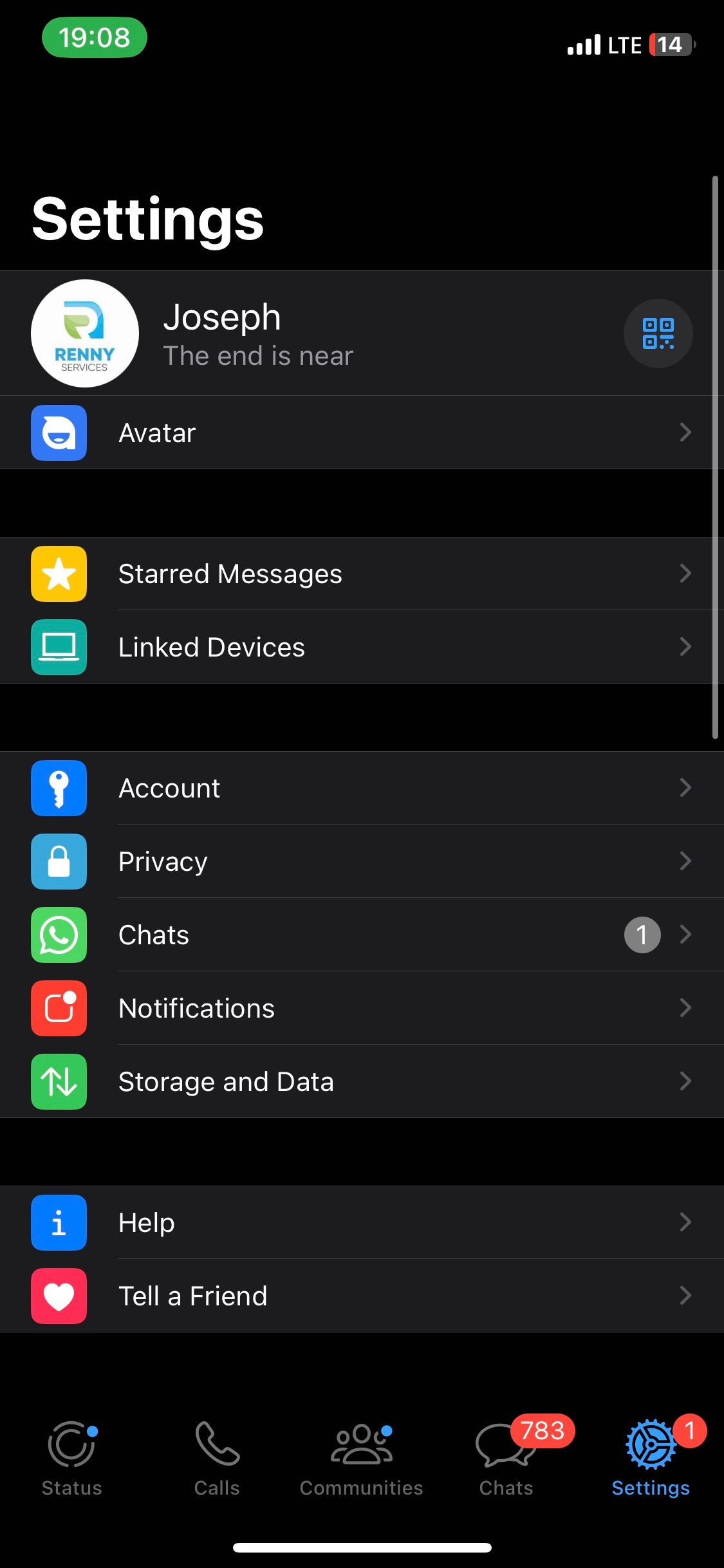This is an image of a mobile phone settings screen displaying a variety of options and status indicators. The background is black with mostly white text. 

In the upper left-hand corner, a curved green rectangle with "1908" in white text is visible. To the upper right-hand corner, there are four bars representing mobile signal strength labeled as LTE, next to a slightly blurred red icon with the number "14" on it, possibly indicating notifications.

At the top of the screen in large white text, "Settings" is written, followed by "Joseph." Beside "Joseph" is a small circle containing tiny, unreadable text in colors blue, green, and red. Beneath Joseph’s name, a phrase, "The end is near," is displayed. On the far right is another circle with four small blue squares inside.

Below this heading, various settings options are listed:
1. **Avatar**: Accompanied by a blue square with what appears to be a planet image.
2. **Shared messages**: A square with a star against a yellow background.
3. **Account**: Displayed with a blue square icon featuring a white key.
4. **Privacy**: Indicated by a lighter blue square with a white padlock.
5. **Chats**: A green square with a phone icon resembling WhatsApp's icon.
6. **Notifications**: Represented by a red icon with a white square and a small bubble.
7. **Storage and Data**: Marked with green up and down arrows.
8. **Help**: Shown with a blue background and an eye icon.
9. **Tell a Friend**: A white heart on a red background.

At the bottom of the screen, there are navigation icons for Status, Calls, Communities, Chats, and Settings. Both Status and Communities have a small dot above them, while the Chats icon shows 783 messages. The Settings icon is highlighted in blue with one new message indicator.